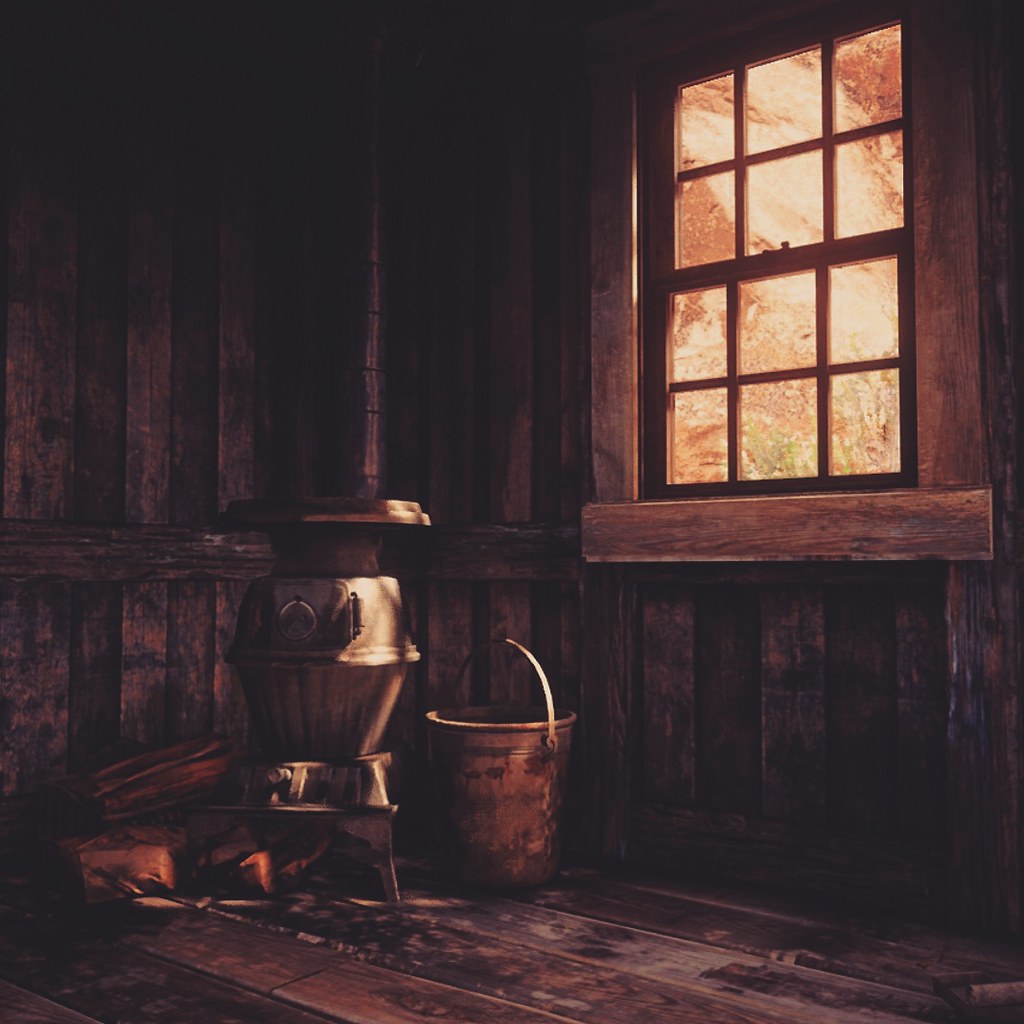This detailed depiction presents an interior view of an old wooden building, likely a photograph given its unsigned nature. The structure features a weathered wooden wall adorned with a single window consisting of two sashes, each with six small panes separated by thin wooden dividers. Through the glass, a rock wall or brown grassy hill is slightly visible, suggesting a rustic outdoor setting. The floor, composed of wooden panels, spans diagonally from the bottom right toward the left of the frame, lending an angled perspective to the room's layout.

Dominating the center of the room stands an antique wood stove, characterized by its dark brown and black hues. The stove has a robust presence with its legs elevating it from the floor and a prominent black smokestack that ascends out of view. To the left of the stove rests a small pile of firewood, essential for fueling the heater, while a gray bucket or basket is positioned to the right. Despite the crude and aged construction of the space, every element from the wooden slats of the walls to the utilitarian placement of the stove and its accessories speaks to a bygone yet functional living environment. The room is otherwise sparsely furnished, emphasizing the raw, minimalist charm of this rustic dwelling.